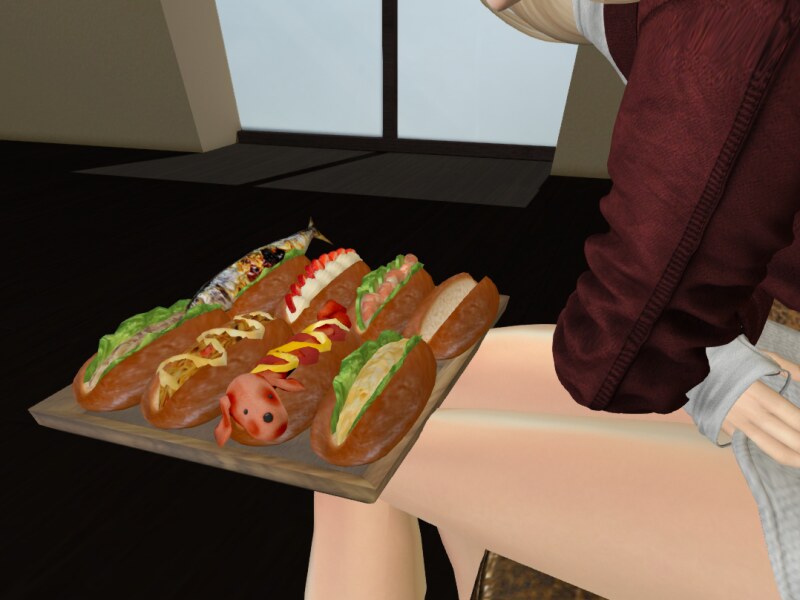The image appears to be a computer-generated or AI-created artwork with a slightly surreal quality. It depicts a scene where a woman, whose head is not visible, is sitting on a black-bottomed floor against a white wall. She is positioned to the right side of the picture, appearing to look out a large, floor-to-ceiling window that is bisected by a black bar. She is clad in a burgundy jacket, a grey-edged top, and short shorts, with either bare legs or tights. Her attire is complemented by a hint of blonde hair and possibly the edge of her chin. In front of her, resting on her knees, is a grey tray with an array of different types of hot dogs or sandwiches, arranged in two layers of four. Interestingly, one of these hot dogs features a tiny toy pig's head, while the rest are adorned with various vegetables and condiments. The overall ambiance of the image is enigmatic, combining elements that make it look both realistic and oddly disjointed.